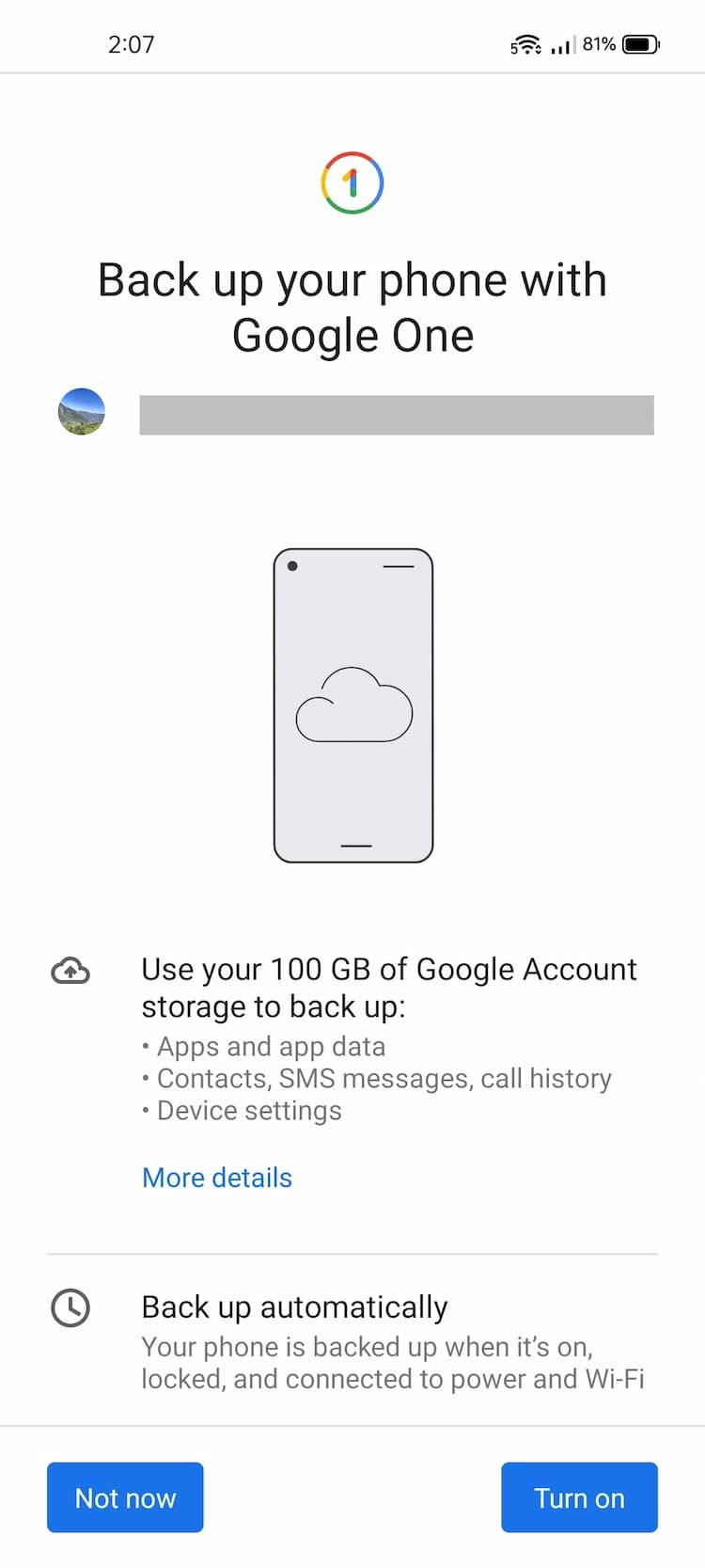A screenshot from a smartphone displays a Google One backup notification, indicating the time as 2:07 with Wi-Fi connectivity and a battery level at 81%. The top of the screen features a colorful circle with the number "1" in the Google colors (red, blue, green, and yellow). Below, the notification reads "Back up your phone with Google One." An illustration of a smartphone screen showing a cloud icon is featured prominently. The text beneath highlights that users can utilize 100 GB of Google account storage to back up apps, app data, contacts, SMS messages, call history, and device settings. It mentions that backups occur automatically when the phone is on, locked, and connected to power and Wi-Fi. Two buttons at the bottom offer the options "Not now" on the left and "Turn on" on the right, both in white text on blue rectangles. The screenshot is portrait-oriented and devoid of any people, animals, plants, vehicles, or aircraft.